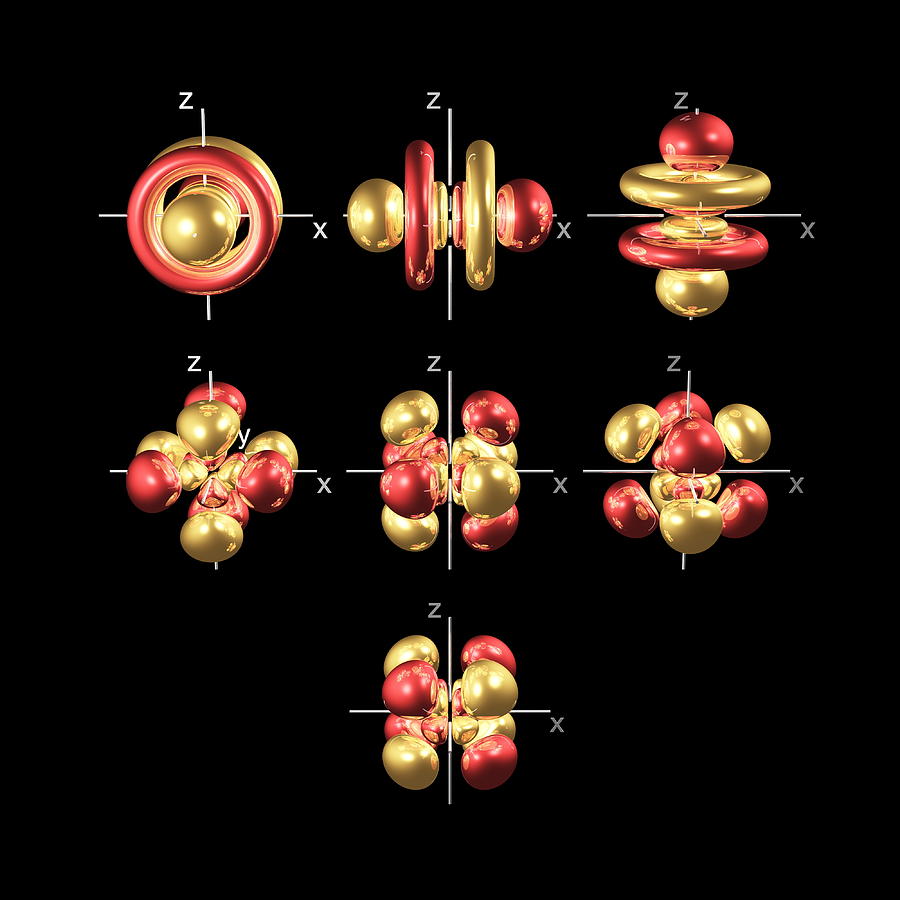The image presents detailed scientific models of atoms or molecules arranged on an X, Y, and Z plane, depicted from multiple perspectives. The black background hosts seven distinct clusters, characterized by interspersed red and gold spheres, highlighted by white crosshairs marked with 'Z' at the top and 'X' to the right, some also bearing a 'Y' label towards the middle. The arrangement features three varied forms: the top row has three structures with red and gold spheres at either end of a rod-like center flanked by large gold and small red rings. The middle row displays three molecules, each as clusters of spherical red and gold portions. At the bottom, a solitary molecule mirrors the clustered form of those in the middle row but is uniquely positioned. Notably, each colored sphere and surrounding rings visually shift based on the perspective, emphasizing the intricate rotational patterns and alignment of the atoms within the model, giving it a layered, teardrop-like appearance.